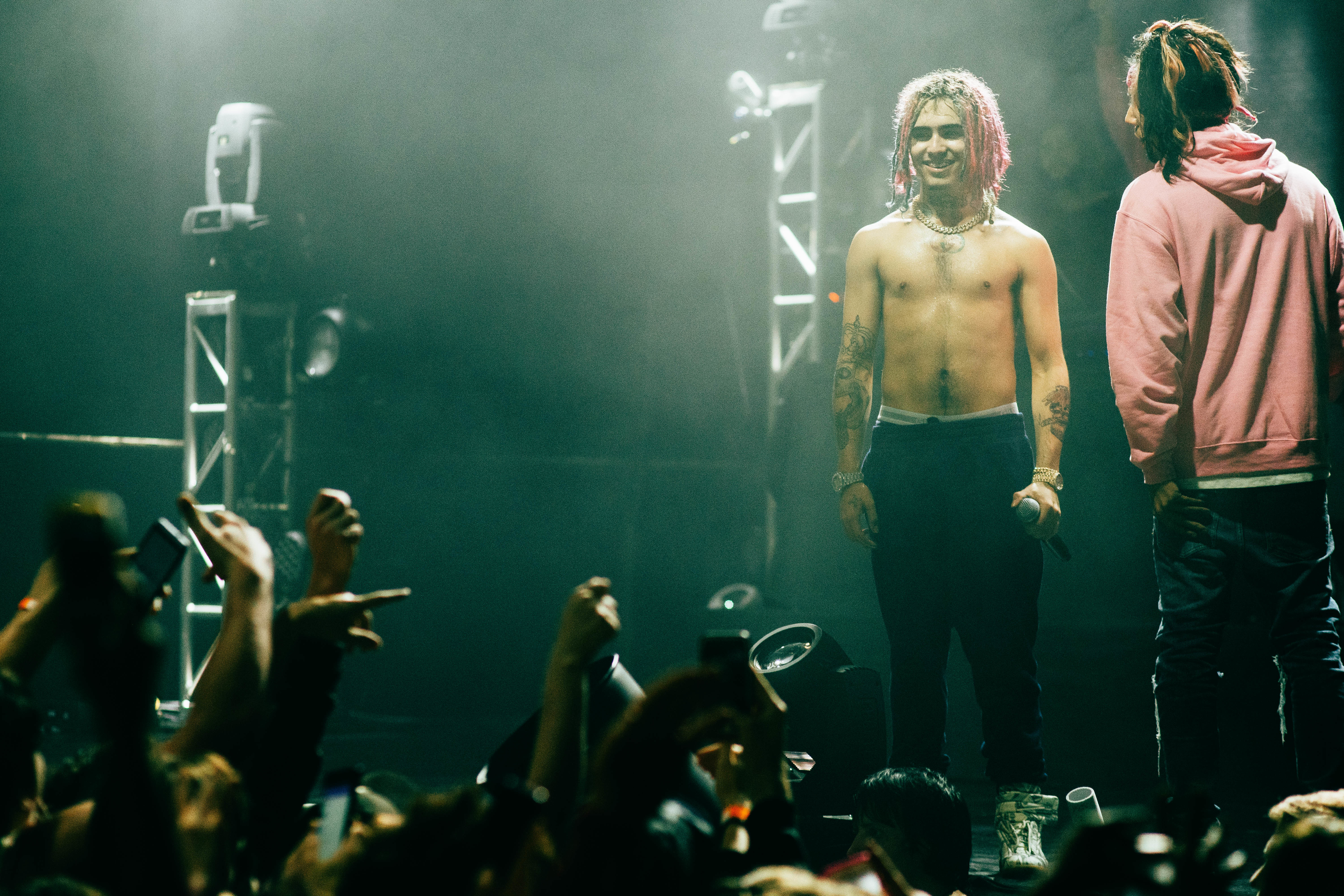The image captures a dimly lit concert scene with a smoky atmosphere, created by a fog machine. In the foreground, the bottom portion of the image shows a crowd of enthusiastic fans with their fists in the air and cameras raised. Overhead, there are vertical spotlight supports casting a hazy glow over the stage. On the right side of the stage, rapper Lil Pump is shirtless, revealing tattoos on his arms and chest, and wearing dark slacks that show the waistband of his undergarments. His long shoulder-length hair is dyed pink, and he holds a wireless microphone in his left hand while grinning at the crowd. To his left, another performer is seen from behind. This individual has dark shoulder-length hair with pink tips, wears a faded pink hoodie, and dark sagging pants. The metal framework for the stage lights is visible in the background, adding to the concert ambiance.